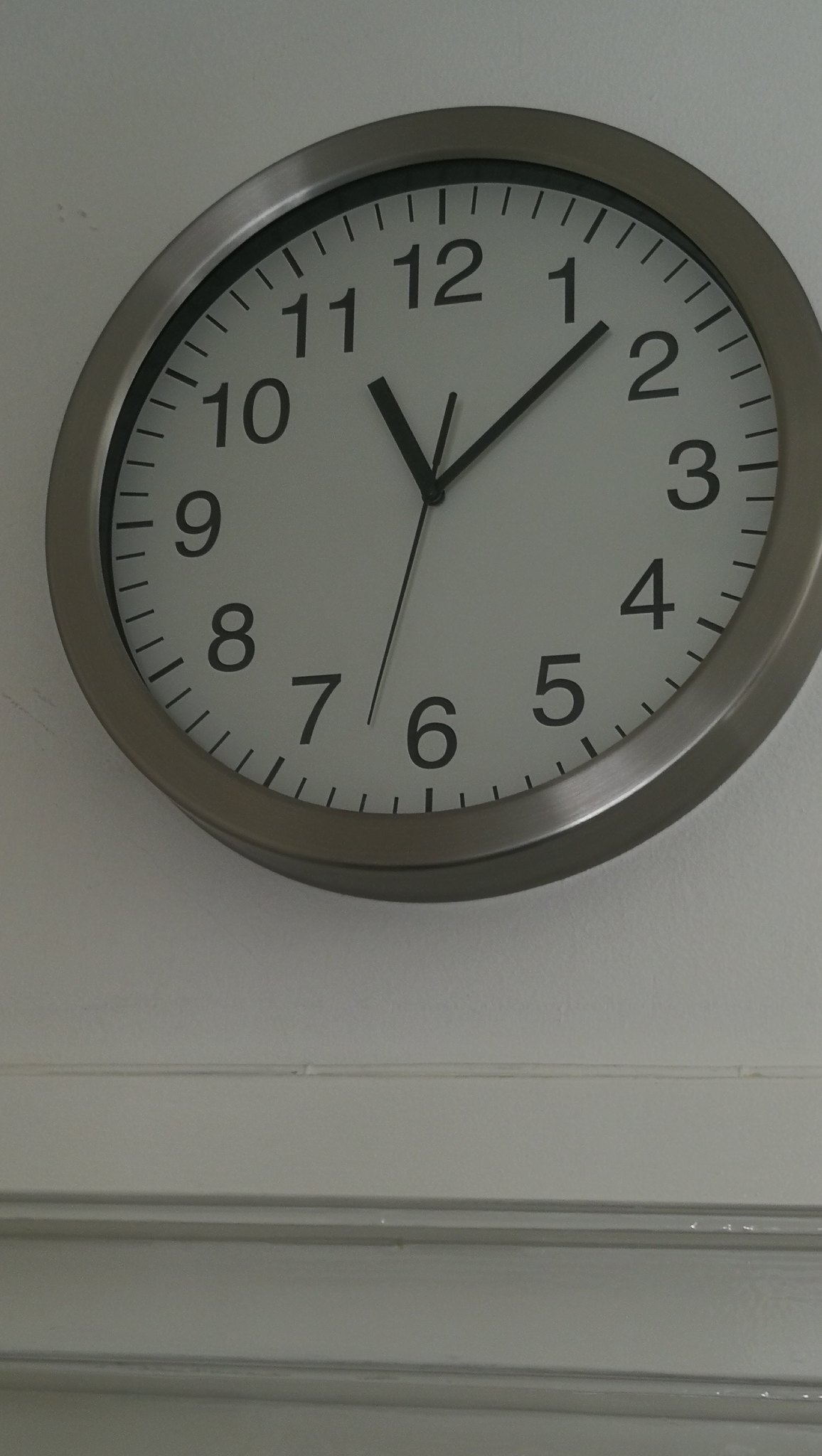A chrome-framed wall clock dominates the upper half of the photograph, set against a pristine white wall with elegant crown molding below it. The molding features two distinct ledges that add a touch of classical refinement to the setting. The clock's face is classic white, with bold black numerals arranged in the conventional sequence from 12 at the top, and slender black minute and hour hands. The time displayed is approximately 11:10 and 37 seconds, with the hour hand pointing towards 11, the minute hand slightly past the 1, and the second hand two ticks past the 6.